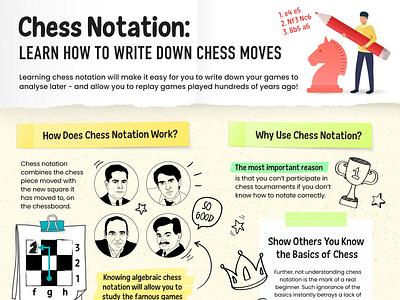The infographic titled "Chess Notation: Learn How to Write Down Chess Moves" serves as an illustrative guide, likely geared towards kids, to help understand the importance and functionality of chess notation. It explains that knowing chess notation will allow players to document their games for later analysis and to replay historic matches. On the top left, the title is prominent in black text set against a white background. Accompanying the title is a clipart of a man in a yellow sweater and blue pants holding a giant salmon-colored pencil, standing next to a large red knight chess piece. Below the title, the section "How Does Chess Notation Work?" describes that chess notation combines the piece moved with its new position on the board. This section is supported by black-and-white portraits of four men, possibly representing chess masters, with their heads depicted in circles. To the right, a blue arrow points through a diagram of a chessboard, and small icons such as a crown and a trophy with the number one further embellish the infographic. The various clipart images, including a scaled-down 3x3 chessboard in the lower left corner, contribute to the engaging, child-friendly design of the guide.